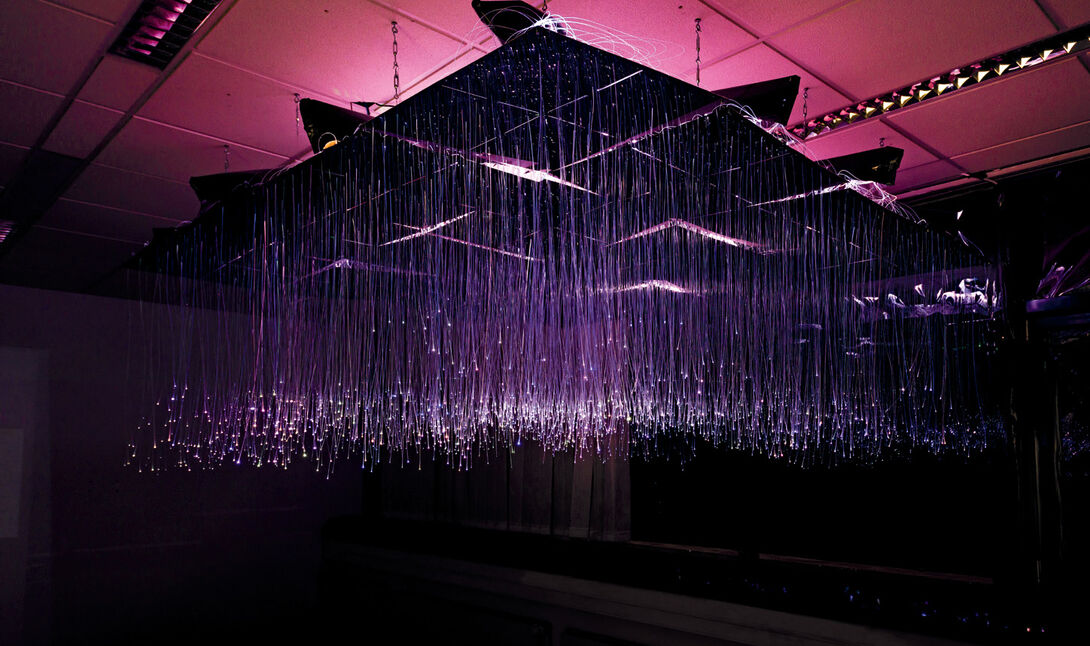The photograph captures an unusual and intricate light fixture hanging from a pink ceiling in a very dark room. The ceiling itself appears red or pink, contrasting sharply against the predominantly dark space. On either side of the image, rows of pink and white studio lights are visible, contributing to the ambient lighting. The central fixture is a striking, multi-layered black installation, somewhat pyramid-shaped with numerous smaller triangular panels. Hanging from this fixture are countless thin, illuminated strands. These strands are predominantly purple, transitioning to white at the tips, evoking the appearance of water streaming down. The bottom of the picture fades into black empty space, further emphasizing the luminous display of the central hanging decoration.